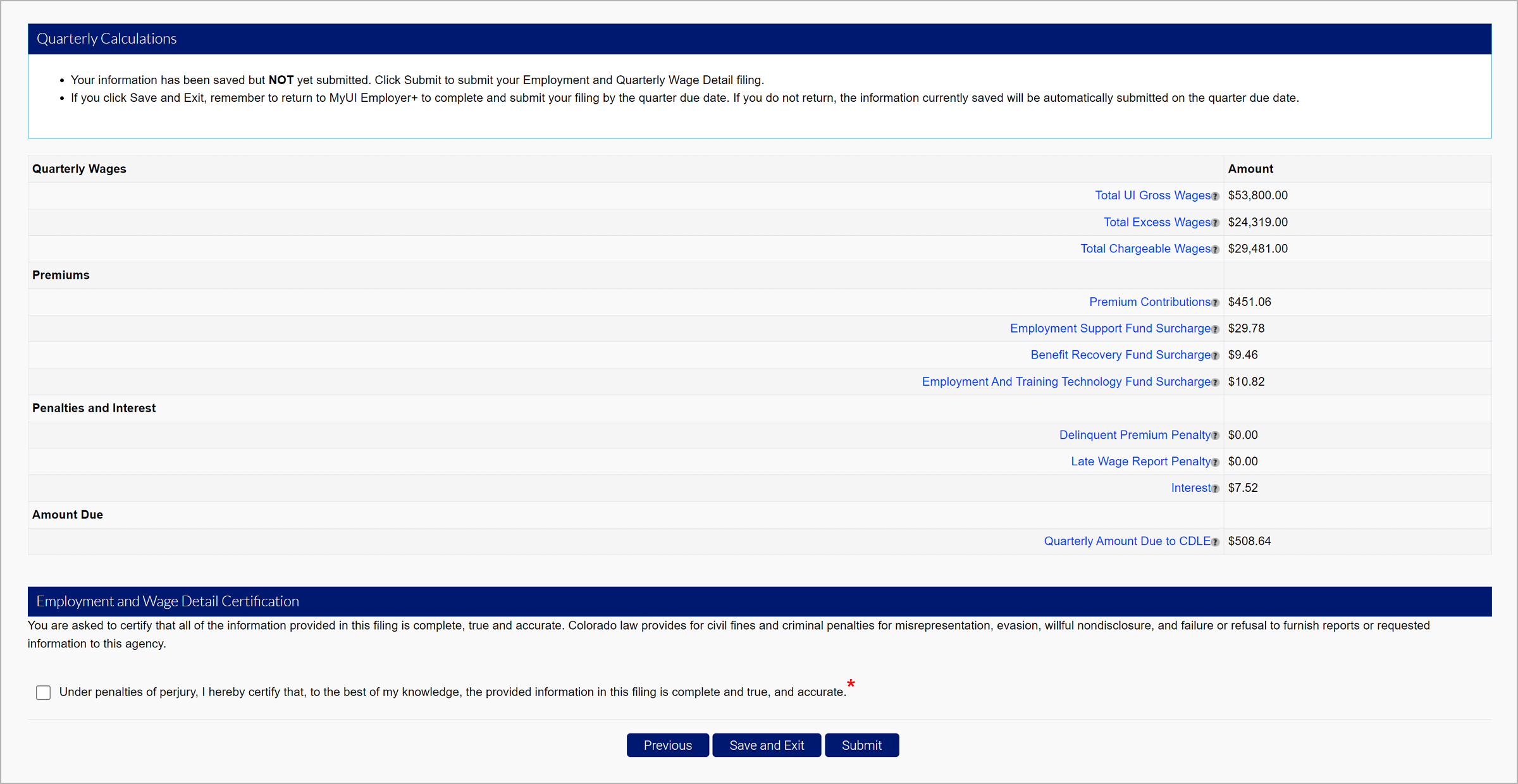This image depicts a webpage designed for employers to submit their quarterly wage and employment details to Colorado’s Department of Labor and Employment (CDLE). At the top of the page, a blue bar is prominently displayed with the header "Quarterly Calculations." Below this header, a notification indicates that the user's information has been saved but not yet submitted. It advises the user to click "Submit" to finalize their employment and quarterly wage detail filing. Should the user choose to "Save and Exit," they are reminded to return to the "My UI Employer" section to complete and submit their filing by the quarter's due date. Failing to do so will result in the information being automatically submitted on the due date.

The webpage provides detailed financial data, including:
- Total UI Gross Wages: $53,800
- Total Excess Wages: $24,319
- Total Chargeable Wages: $29,481
- Premium Contributions: $451.06
- Employment Support Fund Surcharge: $29.78
- Benefit Recovery Fund Surcharge: $9.46
- Employment and Training Technology Fund Surcharge: $10.82
- Delinquent Premium Penalty: $0
- Late Wage Report Penalty: $0
- Interest Cost: $7.52
- Quarterly Amount Due to CDLE: $508.64

At the bottom of the page, there is a section titled "Employment Wage Detail Certificate." Employers are required to verify that all the information provided is complete, true, and accurate. The webpage notes that under Colorado law, misrepresentation, evasion, willful nondisclosure, and failure or refusal to furnish required reports or information can result in civil fines and criminal penalties. There is a checkbox for users to certify under penalties of perjury that the information they have provided is accurate to the best of their knowledge.

The interface also includes three buttons— "Previous," "Save and Exit," and "Submit"— all styled in blue. The majority of the webpage features a clean white background with blue and black text, ensuring readability and clarity.